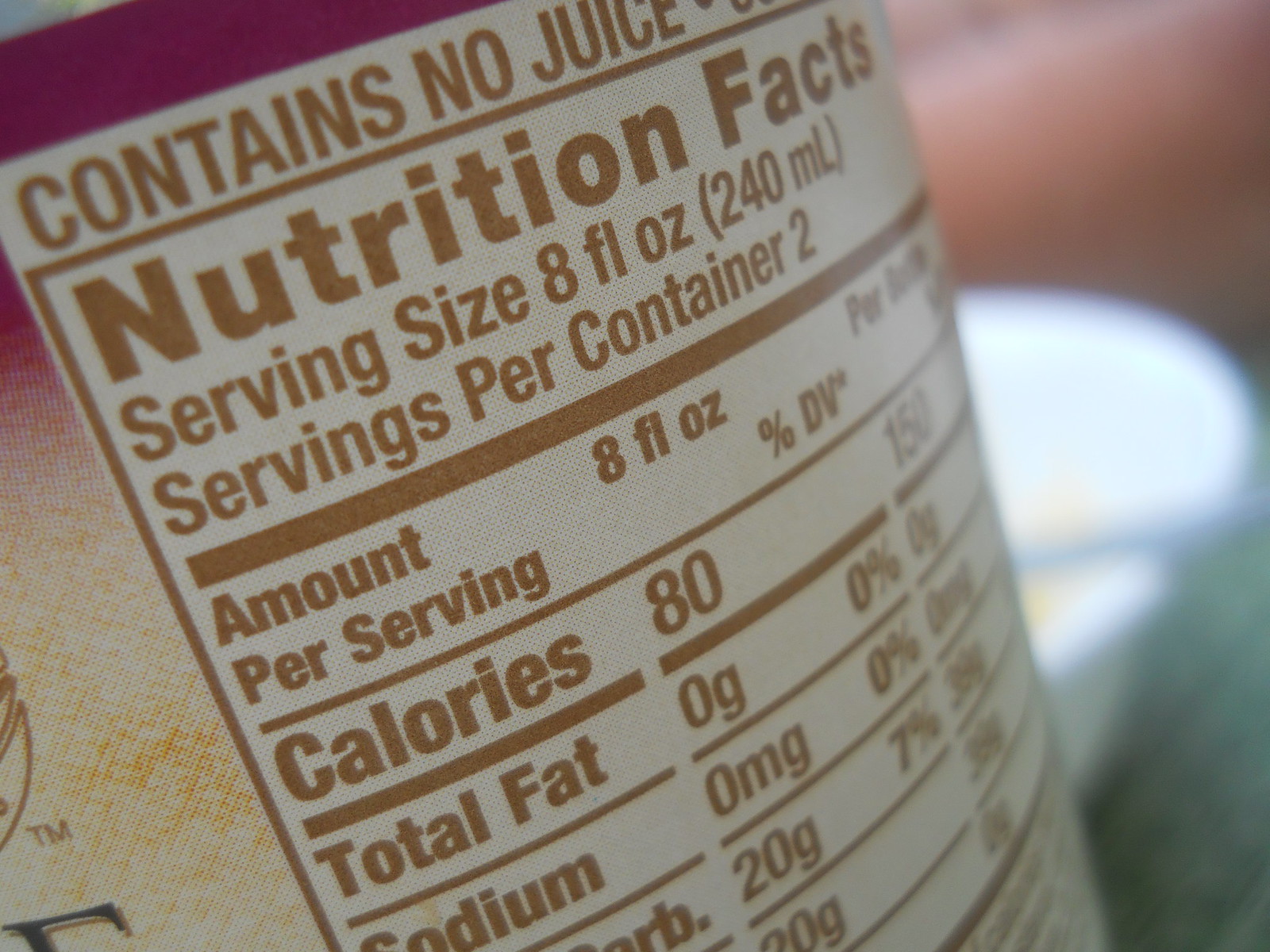This close-up photo captures the partial view of a nutrition facts panel on a can. The label, primarily white with tan writing, emphasizes key nutritional information such as "contains," "serving size: 8 fluid ounces (240 ml)," and "servings per container: 2," along with calories, total fat, sodium, and total carbohydrates. The top part of the label features a pink section that transitions into an orange middle area. On the bottom left, the edge of an 'E' can be seen, and on the top right, there's a faint outline of something white, possibly a bowl with a spoon blurred in the greenish background. The words are inscribed in gold, adding a distinctive touch to the label’s aesthetic.